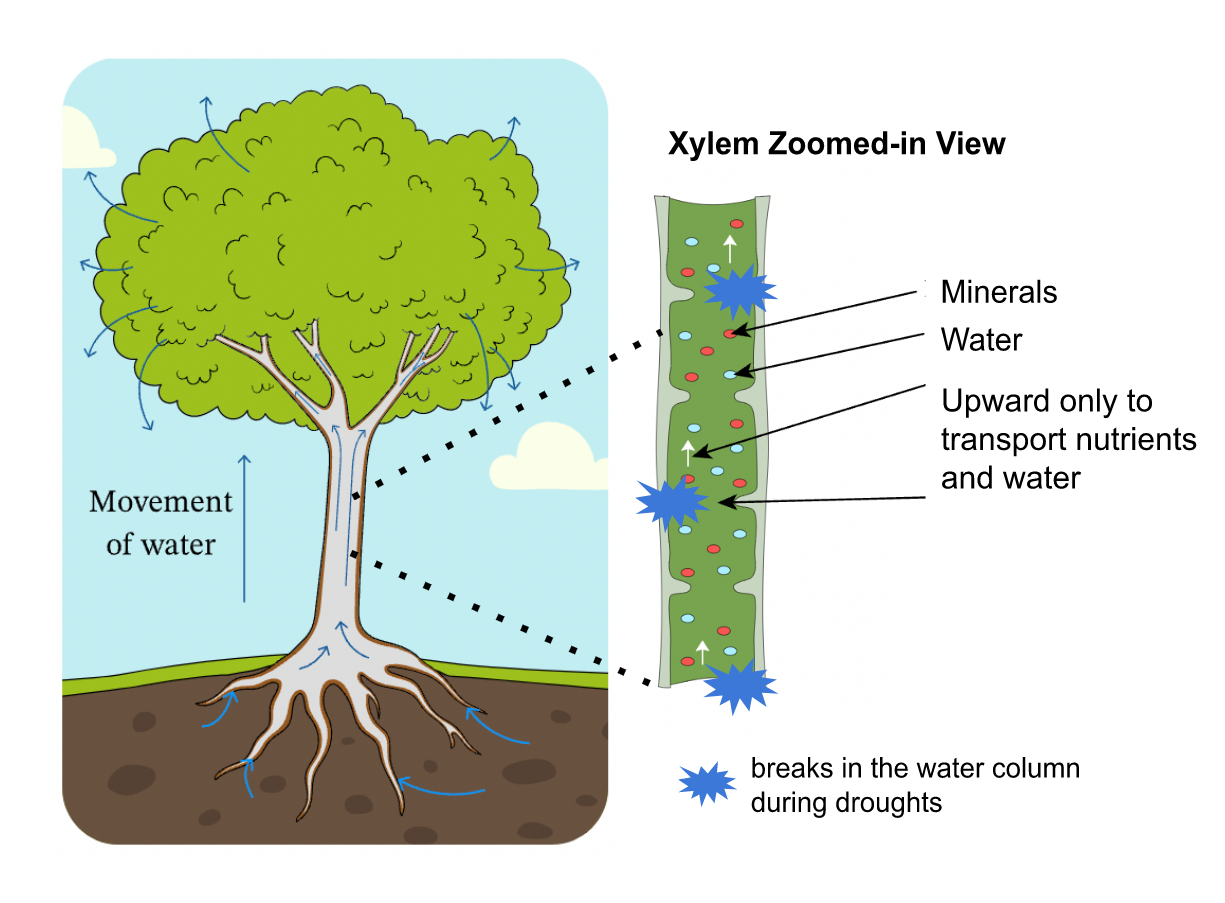The image is an educational diagram, likely found in a biology or geology textbook, illustrating the water movement within a tree. The diagram is divided into two interconnected sections. The left section features a light blue sky background with a cartoon-like tree. The tree has light green leaves and a white trunk with roots spreading into the brown soil at the bottom. Blue arrows are shown traveling from the roots through the trunk and into the leaves, indicating the movement of water and minerals from the ground upwards. Text alongside this section reads "Movement of Water," and dotted lines connect it to the right section of the image. 

The right section, labeled "Xylem Zoomed in View," presents a detailed close-up. It includes a green tube-like structure with light blue and red dots, symbolizing the transport of water and minerals. Arrows are annotated with terms such as "Minerals," "Water," "Upward Only to Transport Nutrients and Water." There are blue bursts on both the left and bottom areas, labeled "Breaks in the Water Column During Droughts," illustrating potential disruptions in water flow.

Overall, the diagram emphasizes the continuous upward movement of water and nutrients through the xylem from the roots to the leaves, highlighting the process and potential issues during drought conditions.